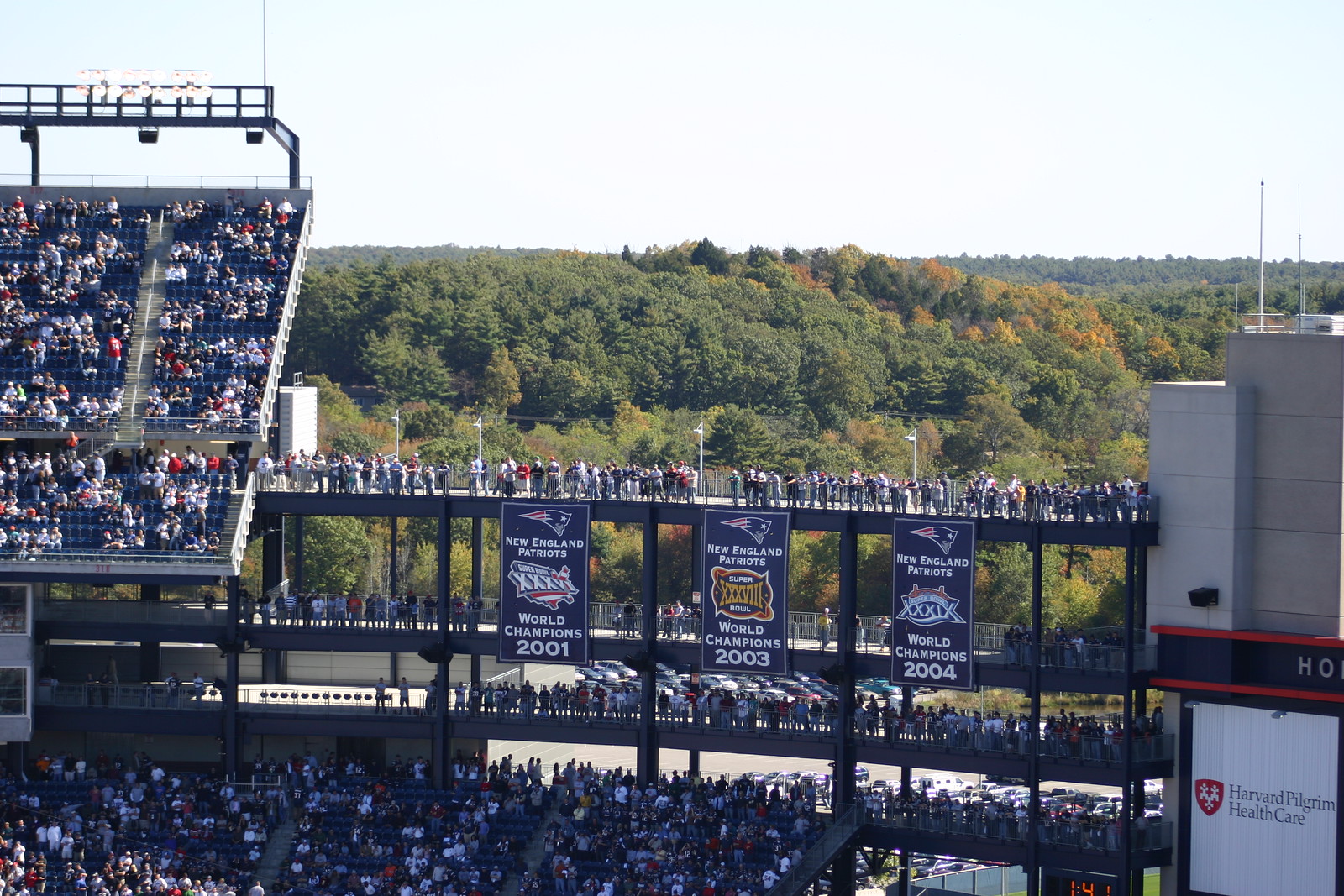This detailed color photograph, taken from a high vantage point in the stands of Gillette Stadium, captures a vibrant scene during a live event where the New England Patriots play. The focal point is the stadium's upper section, which features three prominent banners celebrating the team's World Championships in 2001, 2003, and 2004. These banners hang from catwalks that span across the image from left to right, above a crowded area where fans are standing. Below these catwalks are the main seating areas, filled with thousands of seated fans, extending down to the partially visible lower bowl of the stadium. To the right, a tall cement structure supports an advertisement board for Harvard Pilgrim Health Care. The top of the image shows a light bar illuminating the scene. On the left, the stands rise steeply and are packed with spectators. In the background, a large forested area with deciduous trees, some beginning to turn orange and yellow, stretches out, indicating the early fall season. The clear blue sky above enhances the outdoor setting of this lively sports event.